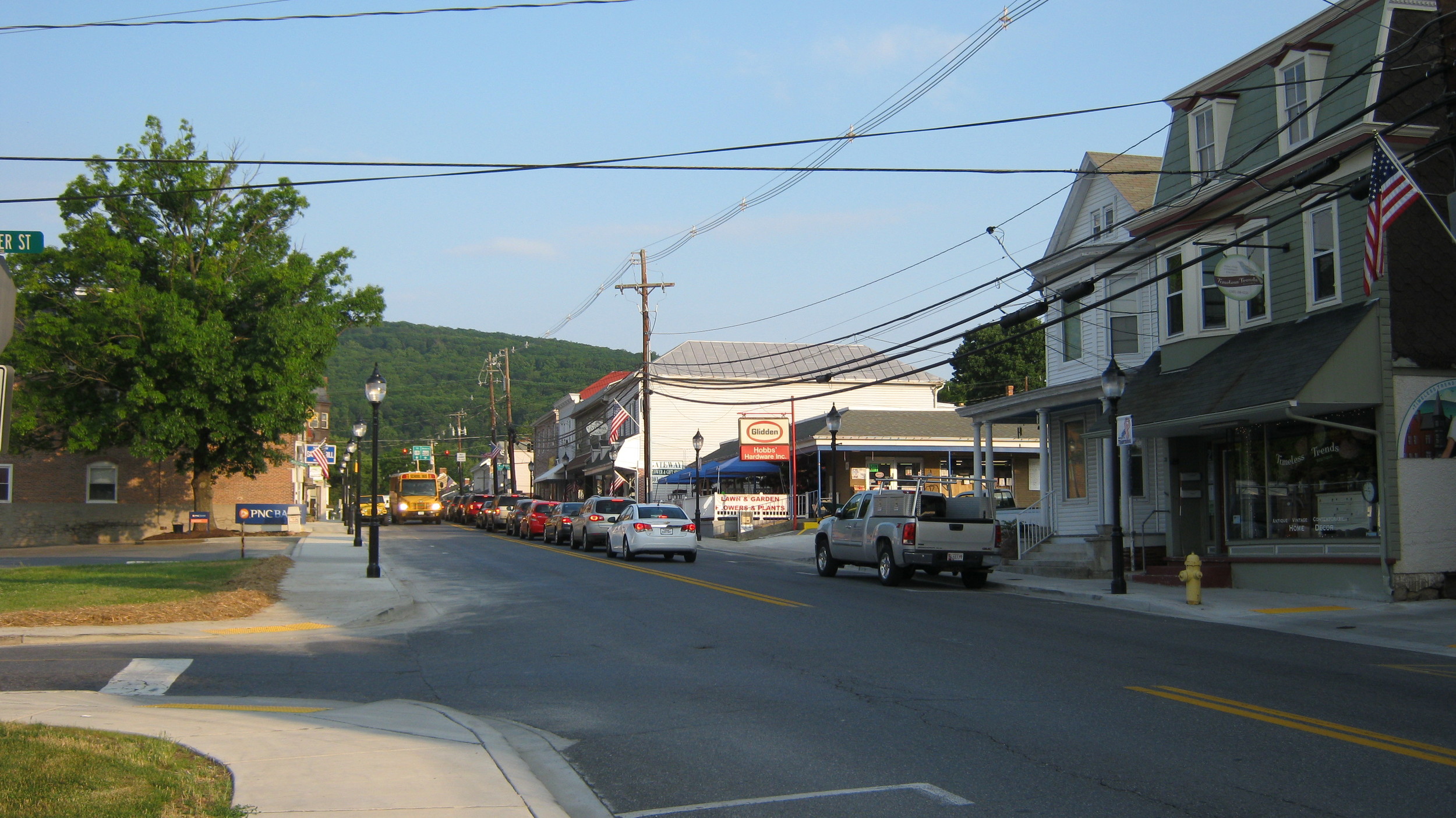The photograph depicts a small American town during what appears to be either late afternoon or early evening, as indicated by the length and direction of the shadows. The image showcases a bustling intersection with a yellow broken-lined street forming a T-junction. On the left side of the image, there is visible foliage from a large tree with leaves, accompanied by a PNC Bank building and a partially visible street sign that reads "R Street." Adjacent to this area stands a brick building, and further along, a yellow bus approaches from afar.

The right side of the image is marked by a variety of buildings and businesses, including a light green three-story structure which seems to serve as both a store and residence. Additionally, there is a white building that might be a hardware store. The street is lined with numerous cars stuck in traffic, their brake lights glowing red, and a parked truck nearby. Overhead, an array of telephone poles and power lines stretch across the top of the image, some adorned with American flags. 

In the background, majestic mountains loom over the horizon, adding a picturesque quality to the scene. The ground-level view captures a yellow fire hydrant and concrete sidewalks, weaving together the quintessential components of a small, vibrant American town.